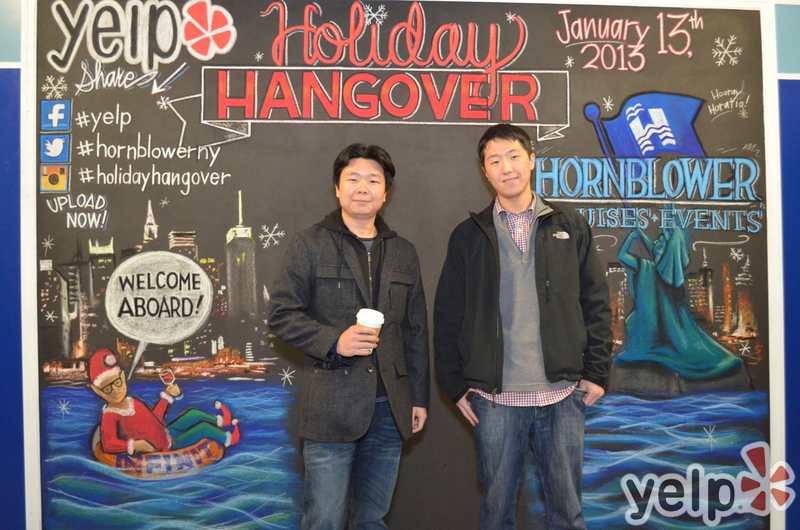In this landscape-oriented photo, two Asian gentlemen stand side by side, both dressed casually in blue jeans. The man on the left sports a dark blazer jacket hybrid and holds a coffee cup in his right hand. He has dark hair and his left hand hangs by his side. The man on the right wears a North Face shell jacket over a gray sweater and a plaid shirt, with his left thumb tucked into his front pocket and his right hand resting by his side. Both are standing in front of a large gray billboard featuring intricate chalk art. 

The chalkboard display is vibrant, showcasing a quirky depiction of the New York City skyline with notable details such as an altered Statue of Liberty and a Santa's elf floating on an inflatable donut, yelling "Welcome aboard." At the top left corner, the recognizable Yelp logo is visible, with social media icons for Facebook, Twitter, and Instagram running down the left edge. Prominently displayed in the center are the words "Holiday Hangover" in red, indicative of a festive or post-holiday celebration event possibly hosted by Yelp, evident by the presence of two Yelp logos at the top left and bottom right corners. Further confirming the event details, the right side of the billboard mentions "Hornblower Cruises and Events" along with the date January 13, 2013. The hashtags #HolidayHangover and #HornblowerNY further tie the scene to a New York-themed holiday event.